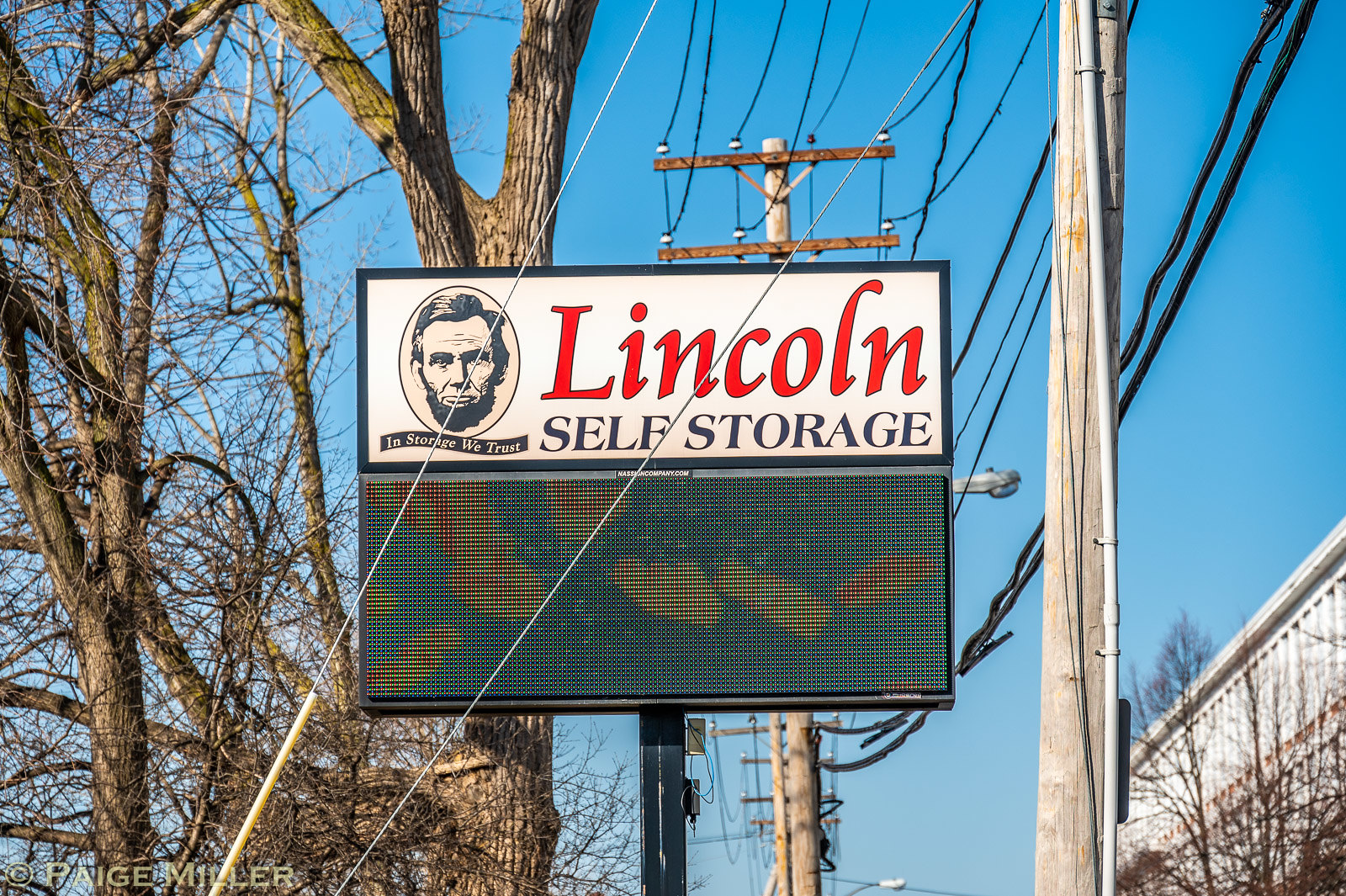The photograph is a horizontal rectangular image capturing a business sign at the center. The top part of the sign features a white band with the text "Lincoln" in red letters, and below it, "self storage" in black letters. To the left of this text is an image of Abraham Lincoln, with an unreadable banner under his face. Underneath this segment, there's a design or symbol that is not clearly identifiable. The background of the picture includes power poles to the right, with one being partially obscured by the sign. On the left side, there are trees, and two wires which might be supporting the power pole cross over the sign. In the lower right corner, there's a visible building. Additionally, a digital sign is present below the main sign, but it appears to be unlit. Several power lines of varying thickness stretch from the top right corner towards the middle of the image.